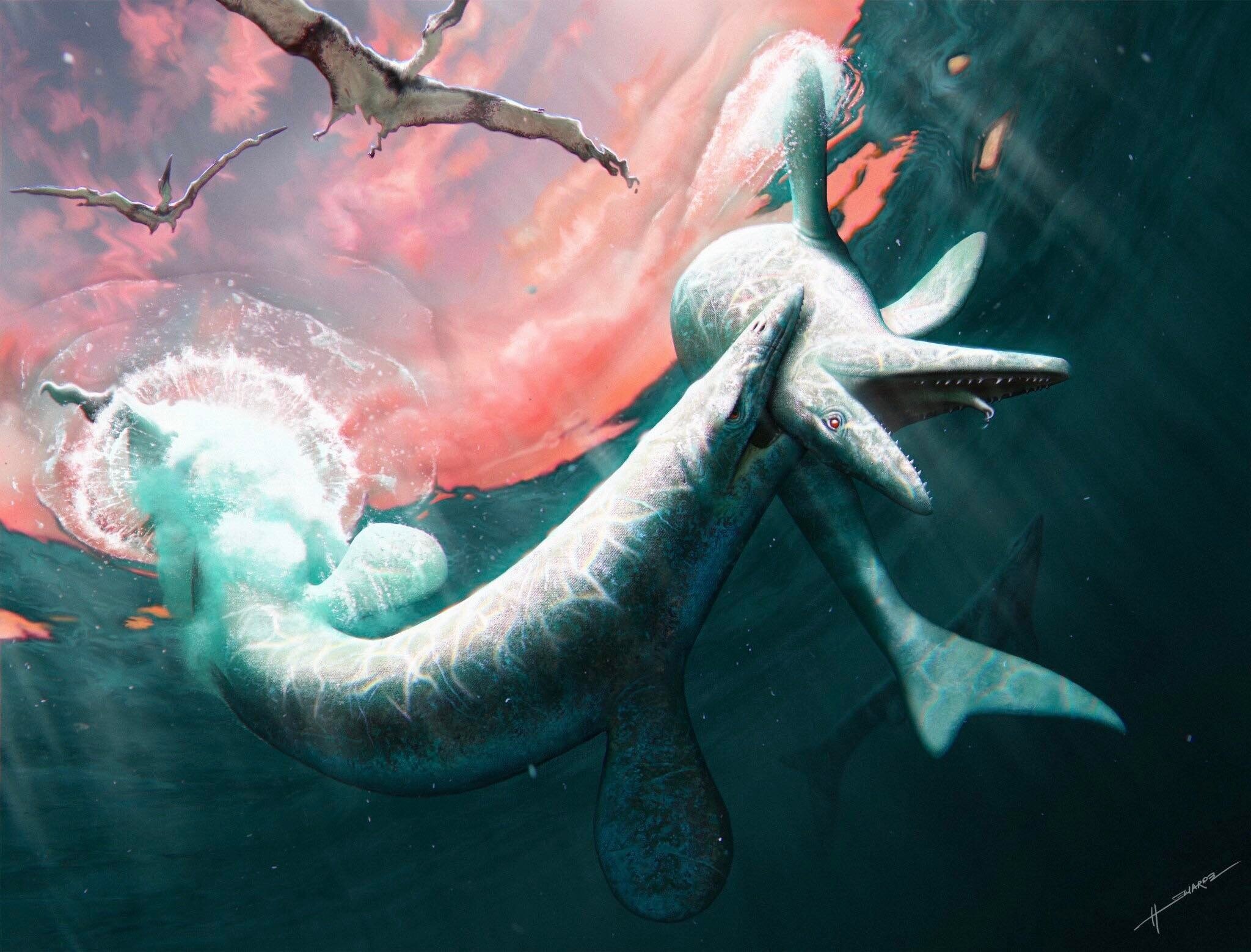This detailed computer-animated image depicts a vivid scene from a prehistoric era, featuring two interacting dolphins that resemble ancient marine creatures. One of the dolphins is aggressively biting the neck of the other, displaying sharp teeth and an angry expression, with its eyes wide open. The attacked dolphin looks visibly uncomfortable. Part of the tail of the biting dolphin breaks the water's surface. In the background, another dolphin-like creature is seen swimming calmly.

Above the water, prehistoric birds that resemble pterodactyls soar in the sky, which is beautifully streaked with shades of pink and blue. Their wings are stretched wide, adding to the dynamic nature of the scene. The image, possibly a digital painting or drawing, is signed in the bottom right corner, though the signature is difficult to decipher. The entire composition is brightly colored and crisp, with a clear and naturally lit setting, enhancing the prehistoric ambiance that transports viewers back to the age of dinosaurs.